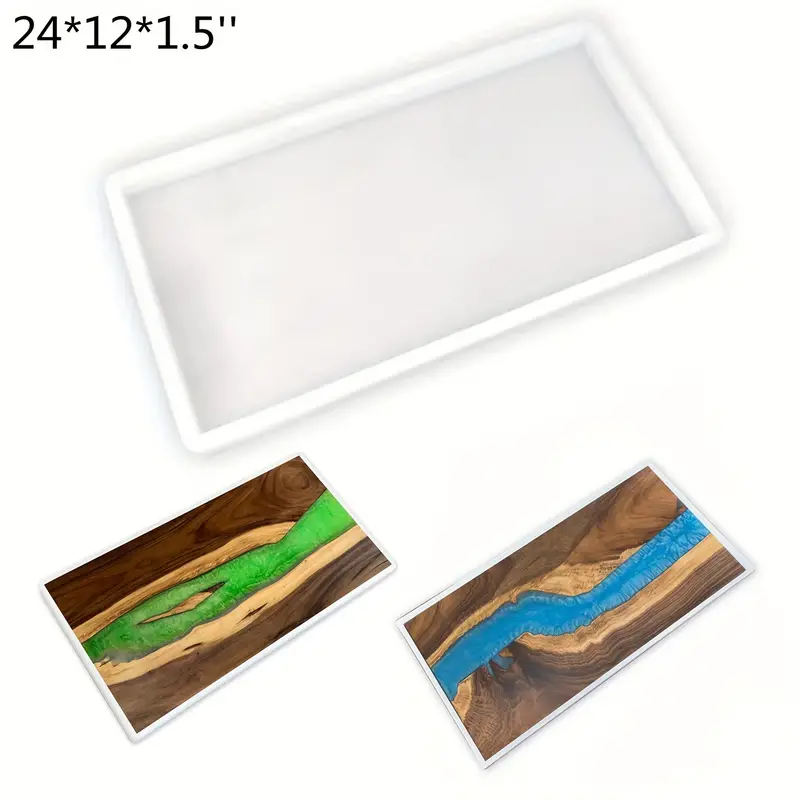The image depicts a white silicone mold intended for resin work, shown against a white background. At the top of the image, black text displays the dimensions "24 * 12 * 1.5 inches." Directly beneath this text, an empty white tray, horizontal in nature, is pictured. Below this empty tray, two examples illustrate the mold in use: the left-hand example features a dark brown wooden piece with green resin filling, bordered by a matching white frame, while the right-hand example displays a similar wooden piece filled with blue resin, also within a white frame. These examples effectively demonstrate potential creative applications for the mold by showcasing how differently colored resins can be used to fill wooden inlays, mimicking natural patterns or designs.